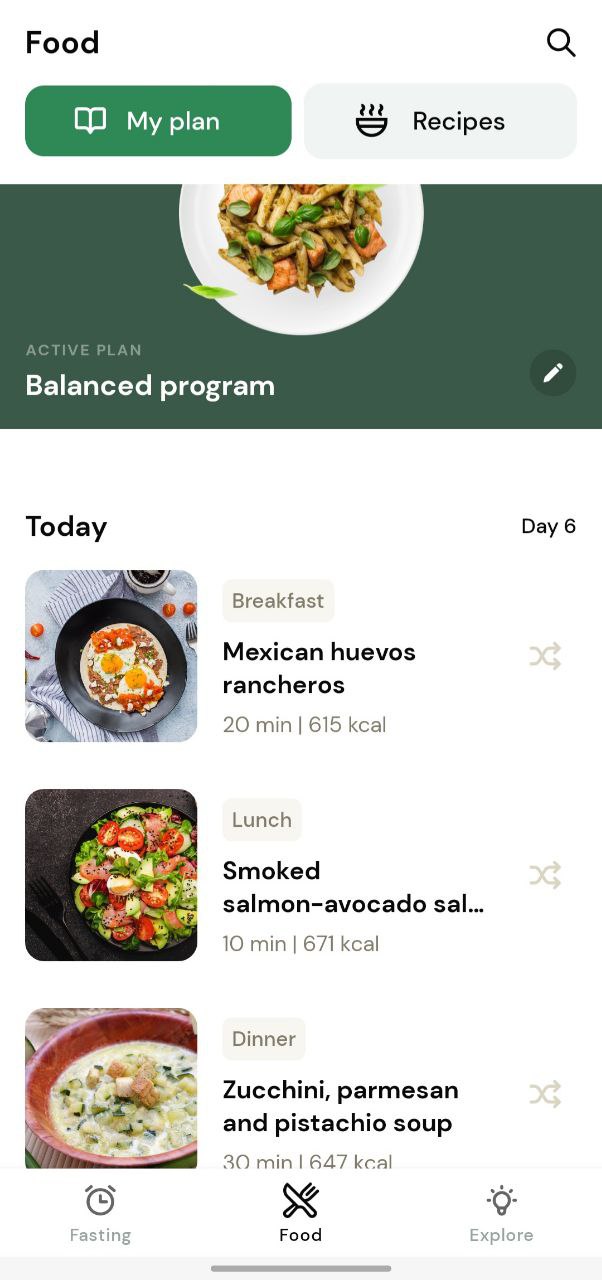Here is a detailed, cleaned-up description of the screenshot:

The screenshot features a food plan interface displayed on a white background. In the top left corner, "Food" is prominently written in black text. On the top right side, there is an hourglass icon. Directly below this are two horizontal rectangles; the one on the left is green with an icon of an open book and the text "My Plan," while the one on the right is gray with an icon of a bowl emitting steam and the text "Recipes."

Beneath these rectangles is another green rectangle displaying an image of a white plate containing a mixture of brown, green, and orange food. The phrase "Active Plan" is written in gray text overlaying this image, with "Balance Program" indicated in white text. In the bottom right corner of this section is a circular icon resembling a location pin.

Further down, the text "Today" is shown prominently on the white background with "Day 6" to its right. Below these headings, there is an image of a black plate featuring a dish that looks like eggs in shades of yellow or orange, accompanied by red and brown accents. This dish is titled "Mexican Huevos Rancheros" and details that it takes 20 minutes to prepare and contains 615 calories.

Following this, a section labeled "Lunch" displays an image of a black plate with red tomatoes and green vegetables, and describes the meal as "Smoked Salmon Avocado Salad," which is ready in 10 minutes and contains 671 calories.

At the bottom of the screenshot, the "Dinner" section showcases a bowl of white soup served in a red bowl, titled "Zucchini Parmesan and Pistachio Soup."

Finally, there are three icons at the bottom: an alarm clock symbol indicating "Fasting," a black knife and fork representing "Food," and a light bulb symbolizing "Explore."